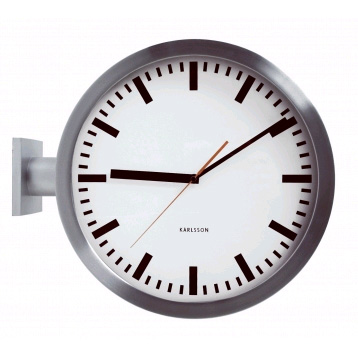The image features an industrial-style Carlson analog clock mounted perpendicularly to a wall, allowing for enhanced visibility from multiple angles. This distinctive clock eschews traditional numeric markers, opting instead for thick, minimalist hour indices. The clock's design includes black hour and minute hands, complemented by a contrasting white second hand. Encased in a sleek silver frame, the clock also features a silver mount that secures it to the wall, enhancing its modern, utilitarian aesthetic.